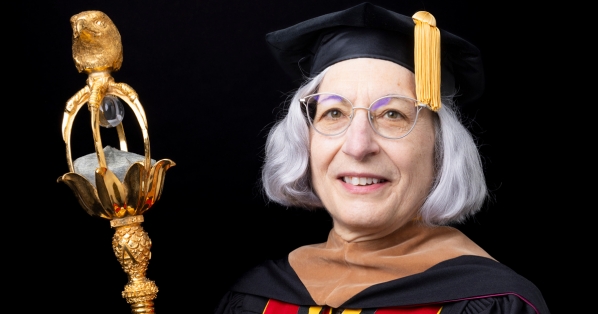In the center of this indoor photograph, set against a solid black background, an older woman is seen smiling warmly into the camera, revealing her upper teeth. She has short, white hair that reaches the length of her neck and wears thin-rimmed glasses, with the golden tassel of her black graduation cap touching the right side of the frame. She is dressed in a black and light brown graduation robe, which features intricate red, black, and yellow details around the neckline. In her hands, she holds an elegant brass or gold staff topped with a golden eagle's head and embellished with a detailed floral design, which includes a white object at its center and legs curving into a cone-shaped base. The staff symbolizes academic accomplishment, and her dignified yet joyful expression reflects her educational achievements.